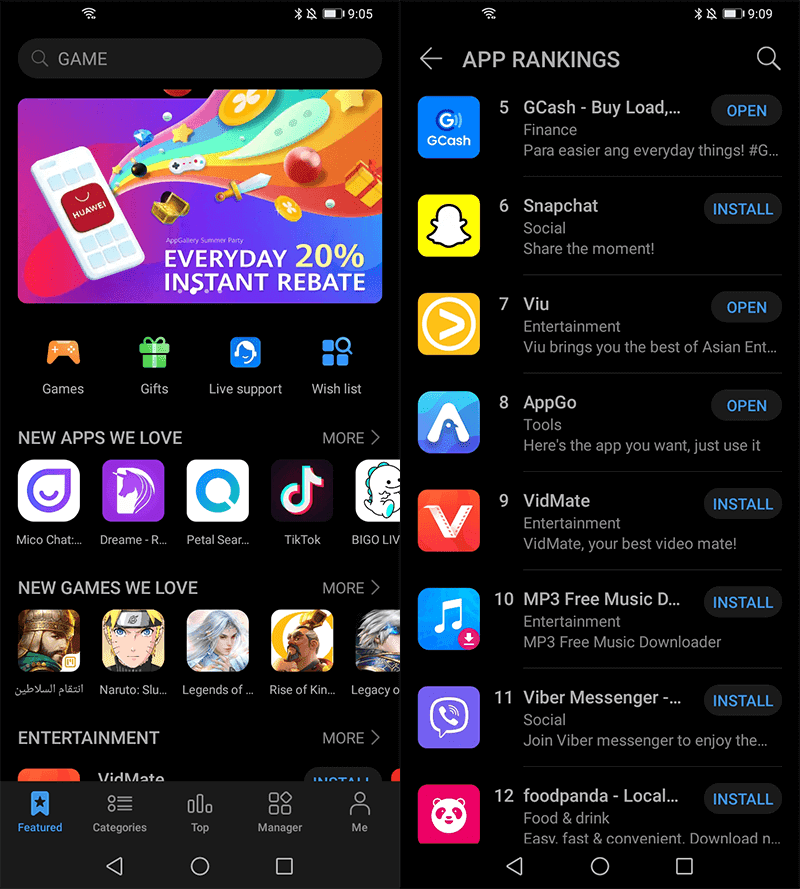### Descriptive Caption

The image features a predominantly black background, presenting itself as a screenshot from a smartphone interface. In the top left corner, there is a search bar bordered in dark gray, containing the word "game" and accompanied by a magnifying glass icon. The status bar at the top of the screen also displays common smartphone indicators, including the current time and battery percentage.

Below the search bar, a vibrant illustration takes center stage. This illustration depicts a smartphone from which an array of rainbow-colored elements is flowing out. Among these colorful waves, various objects are intermingled: a glowing treasure chest, a shiny sword, a gift-wrapped present with a bow, a sparkling star, a speech bubble, and a video game controller. Just beneath this dynamic artwork, text reads "Everyday 20% Instant Rebate."

Further down the screen, four distinct icons are displayed in a row, each representing different categories: Games, Gifts, Live Support, and Wish Lists. Following these icons, the section titled "New Apps We Love" showcases a selection of app names including "My Chat," "Dream," "Pedal Search," "TikTok," and "Bingo Live."

The lower portion of the screen has another section labeled "New Games We Love," featuring a game title written in Arabic script.